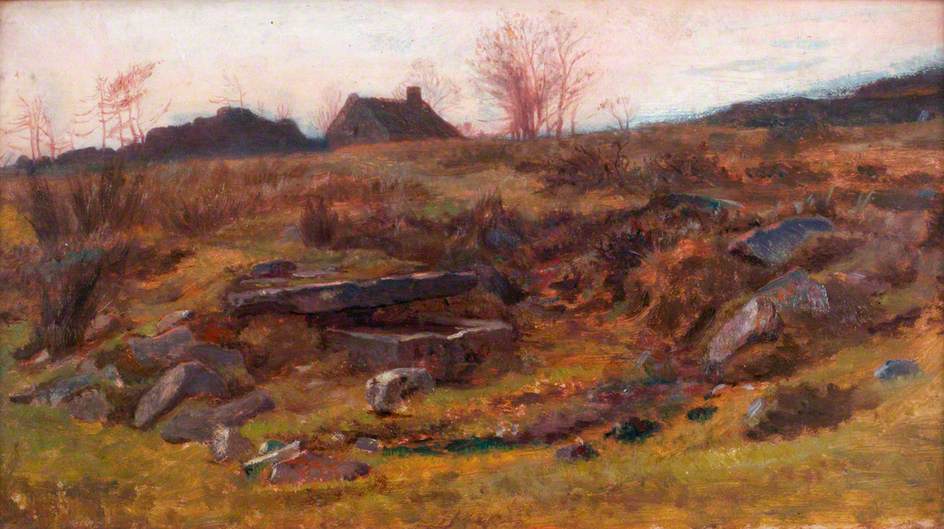The painting is a warm-toned, stylistic watercolor landscape that intricately portrays a rocky and grassy hill. The foreground features an array of golden and yellow grasses, interspersed with dark purples and browns that shift progressively to more browns as the field recedes into the distance. Scattered across the landscape are numerous gray and purplish rocks, adding texture and depth. At the top of the hill, you can see sparse, thin trees alongside a dark brown house with a chimney, situated slightly to the right of center. To the left of the house, large, indistinct masses appear on the horizon, possibly resembling more rocks or additional structures. The sky above is a blend of light pink, blue, and a rusty red, creating an overcast ambiance typical of a serene pastoral scene. The overall composition evokes a tranquil, rustic valley, with no borders or text, allowing the vivid colors and detailed scenery to envelop the viewer fully.